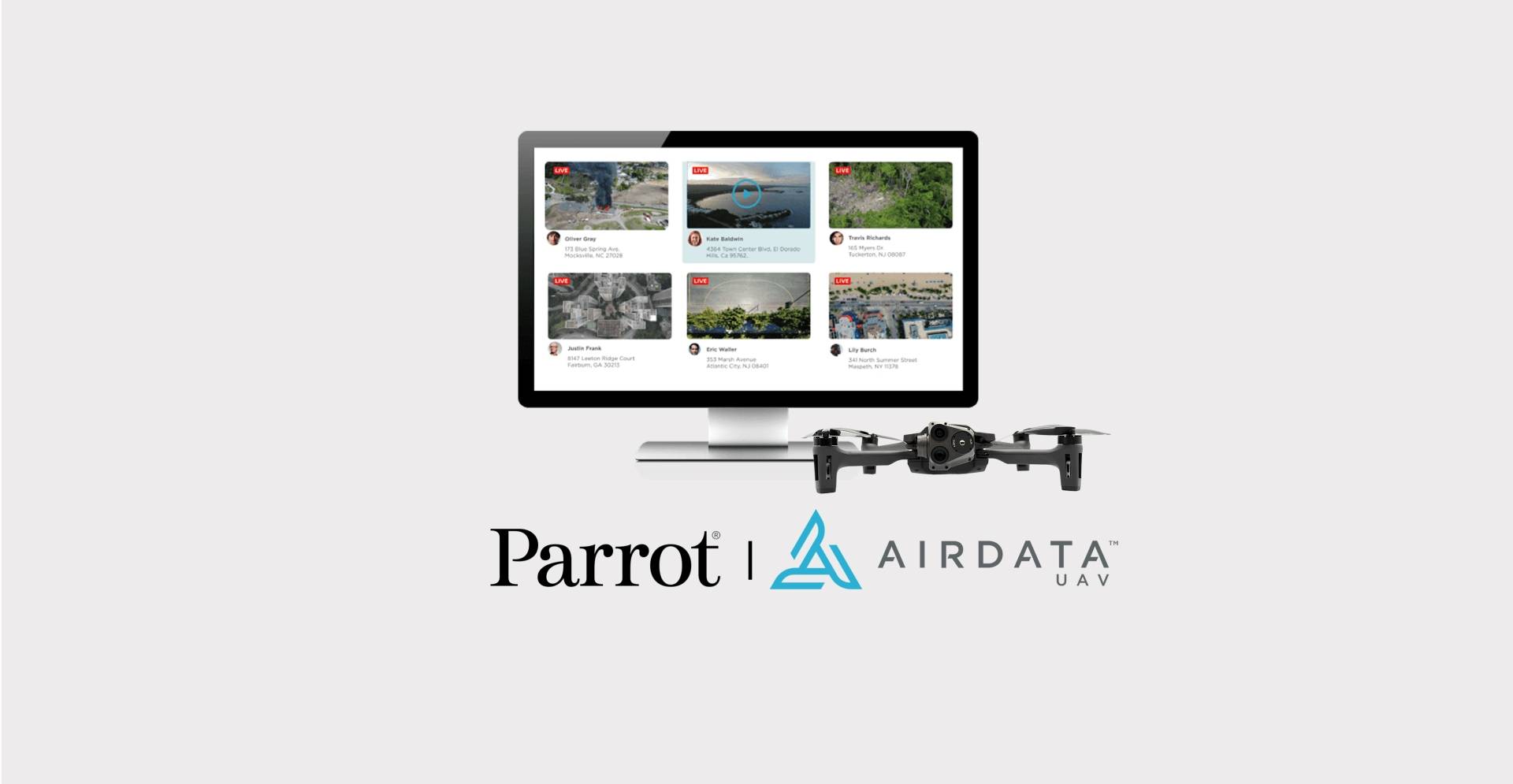The image features a computer monitor with a black frame and a white and silver stand, set against a white background. Displayed on the screen are nine images showcasing various scenes of waterways, trees, and landscapes, likely captured by a drone. In front of the monitor sits a drone with a dark gray and black body, equipped with four propellers. At the bottom of the monitor, black text reads "Parrot," followed by a blue triangle logo, and to the right, the inscription "AirData UAV" in light gray letters.